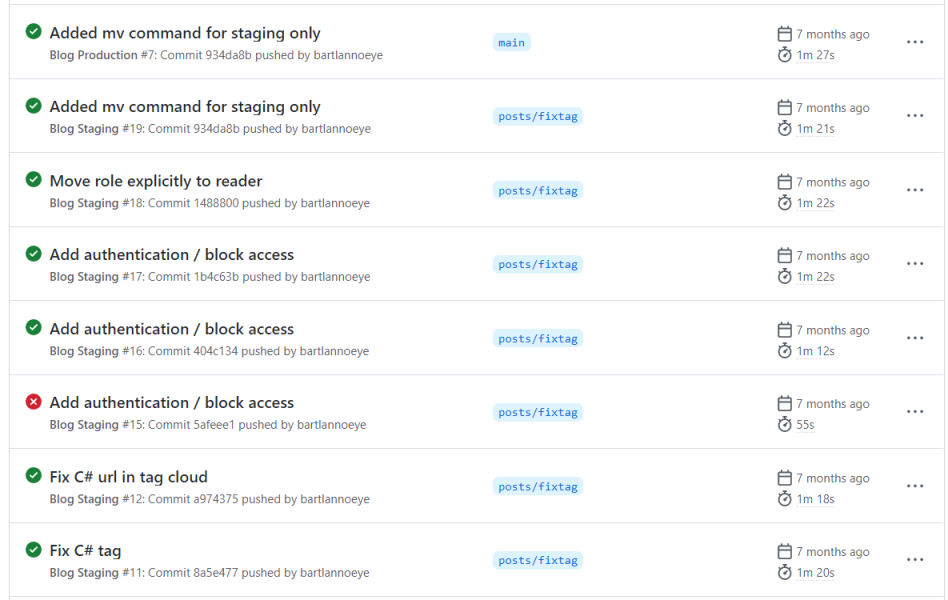The image depicts a command log for a computer system with multiple entries detailing various actions taken over time. Each command is visually demarcated, with some entries marked by green check marks while others have a red X. The background is predominantly white, providing a clean interface for readability. Below is a detailed breakdown of the entries listed in the log:

1. "Add MV command for staging only" - This entry is marked with a green check mark, indicating successful completion. The description includes "Blog production number 7" and states it was pushed by "Bartland OI." This entry is highlighted in blue, denoting its significance. The command was executed 7 months ago and took 1 minute and 27 seconds.

2. Another entry for "Add MV command for staging only" appears, also with a green check mark. The context "Post fix tag" is noted, with the task completed 7 months ago in 1 minute and 21 seconds.

3. "Move role explicitly to reader" - This command is marked with a green check mark. It includes the "Post fix tag" and was executed 7 months ago, taking 1 minute and 22 seconds to complete.

4. "Add authentication. Block access." - Several entries are logged under this description. Some are marked with green check marks, indicating successful completion, and one entry has a red X, indicating a failure or a command that was not executed as desired. These entries vary in execution time, ranging from 55 seconds to 1 minute and 22 seconds, and are all tagged with "Post fix tag."

5. "Fix C number. URL in tag cloud." - This command is marked with a green check mark and also denotes the "Post fix tag." This task was completed 7 months ago and took 1 minute and 18 seconds.

6. Another entry for "Fix C number tag" is marked with a green check mark. Bearing the same "Post fix tag," it was completed 7 months ago in 1 minute and 20 seconds.

Each command is clearly separated and presented on individual lines, making the log easy to read and follow. The overall design is organized and features a mostly white background for clarity.